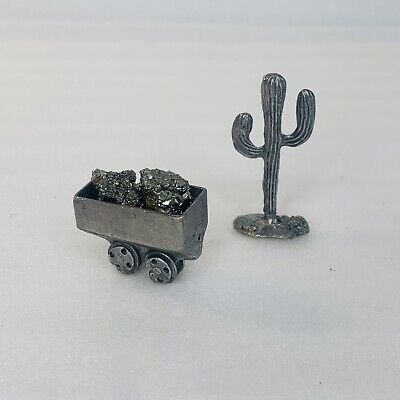The image portrays a monochrome scene featuring two metallic figures placed on an indistinct, light-hued background that fades away toward the edges. On the right, there is a detailed metal casting of a saguaro cactus, characterized by its textured surface with intricate stripes. The cactus has arm-like projections that extend and taper as they join the main body, with the overall figure standing tall and elegant. On the left, slightly lower in position, is a trolley or minecart, rendered in the same metallic material. The cart's design includes two well-defined wheels, each with four holes, and it is filled with rough, craggy chunks that resemble pyrite or gold ore. Together, these figures resemble small tokens, akin to those used in board games like Monopoly, set against a monochrome backdrop with varied black-and-white shadings.